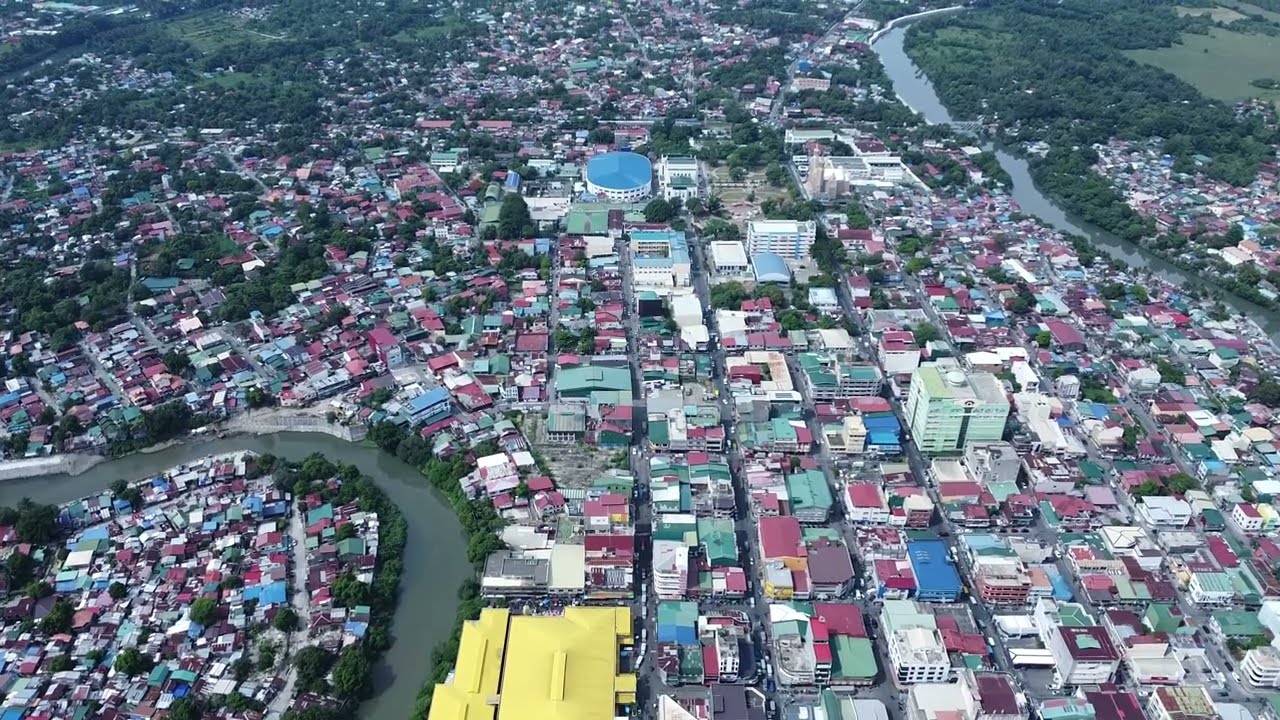The image is a high-altitude aerial view, possibly taken from an aircraft, capturing a densely populated community consisting of various homes, businesses, and taller buildings. The area is vibrant with a mix of colors; the roofs of the structures are primarily green, blue, white, and some purple. Dominating the center of the photo is a tall, light green building that appears to be about eight to nine stories high. Surrounding this central structure, there's an interesting mix of tree-covered areas adding splashes of green amidst the urban landscape. Towards the center-top of the image, a notable round building with a white base and blue roof stands out—possibly a parking deck or sports arena. A prominent river meanders through the city, starting from the upper right, curving around and exiting towards the bottom left. Additionally, near the bottom center, there is a building with a distinct yellow roof. The overall scene is teeming with life, defined by its green spaces intertwined with the urban setup.